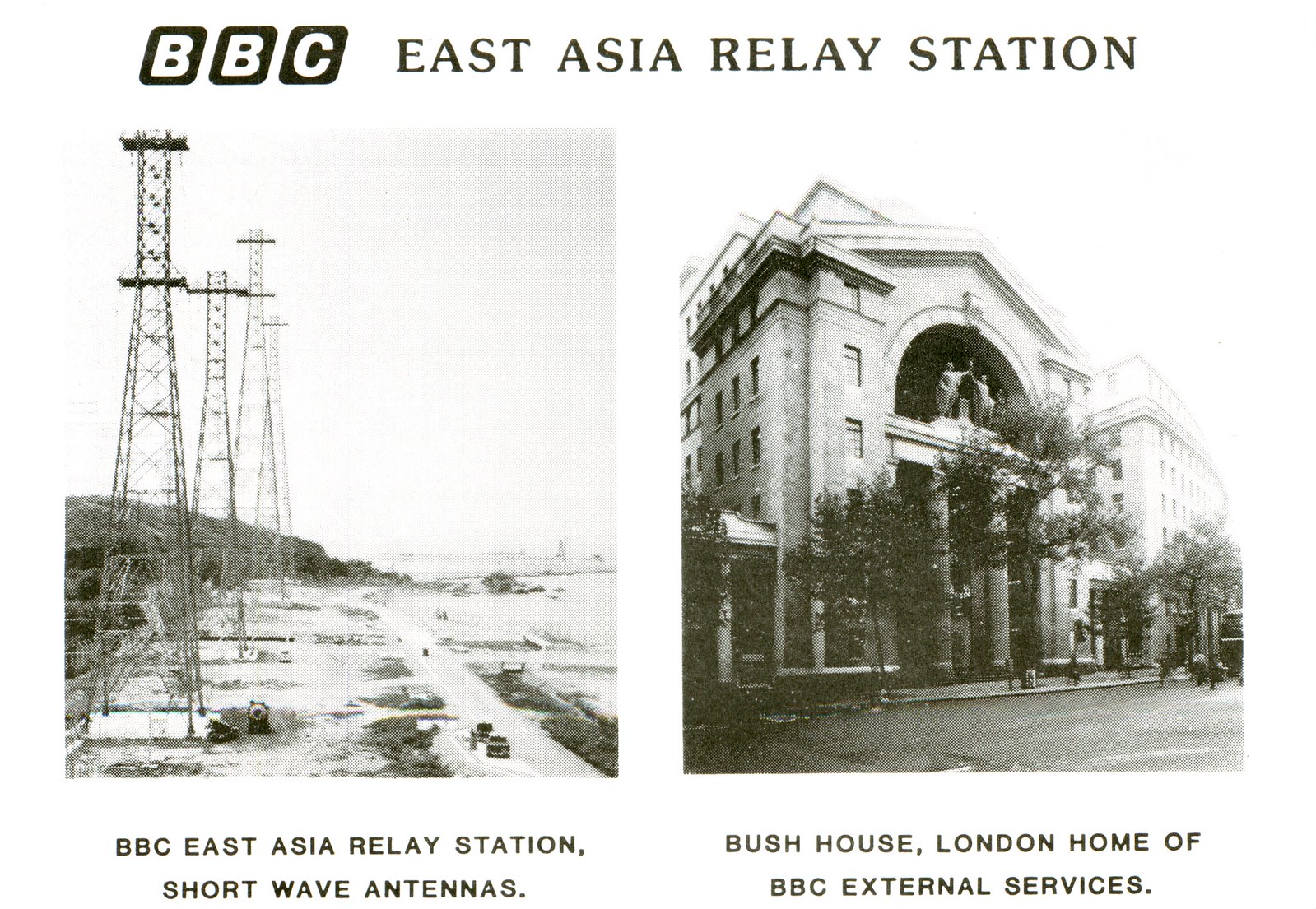The image consists of two black-and-white photographs arranged side by side with a heading above them. The heading reads "BBC East Asia Relay Station."

The left photograph features four towering antennas standing prominently against the sky. Below these antennas, you see a road populated with cars in motion. In the background, there are hills faintly visible, adding depth to the scene. The caption beneath this photo reads "BBC East Asia relay station shortwave antennas."

The right photograph depicts an old, architecturally significant building adorned with statues atop its structure. The scene below the building includes a street lined with several trees and dotted with people walking, adding life to the urban setting. The caption beneath this image states "Bush House London, home of BBC external services."

These carefully composed photographs highlight notable sites associated with the BBC's broadcasting history.